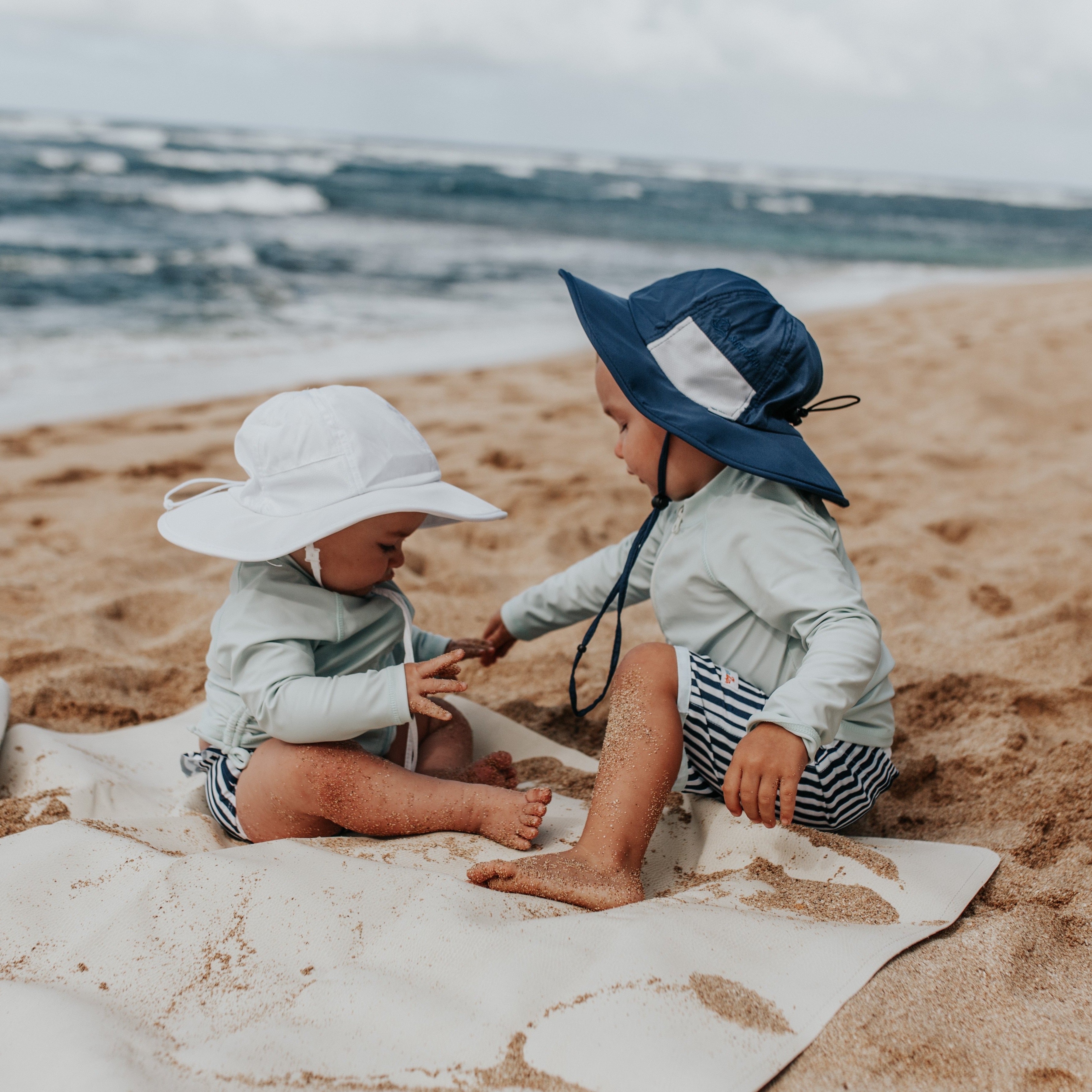In this charming color photograph, two infant siblings—one a baby and the other a toddler—are captured playing joyfully on a sandy beach. They sit on a white blanket that's dusted with sand, exploring the texture with their small fingers. Both children are dressed in matching outfits, featuring dark blue and white striped shorts and light blue-green, long-sleeved tops. The baby sports a white sun hat, while the toddler wears a blue hat with a white patch; both hats are tied snugly under their chins. The backdrop reveals an overcast sky with white clouds and a restless ocean, with waves breaking on the shore. The sandy beach itself has a gentle slope rising from the water's edge. Despite the cloudy sky, the scene is brightly lit, making every detail clear and easy to see, capturing the innocence and joy of the siblings' beach day.